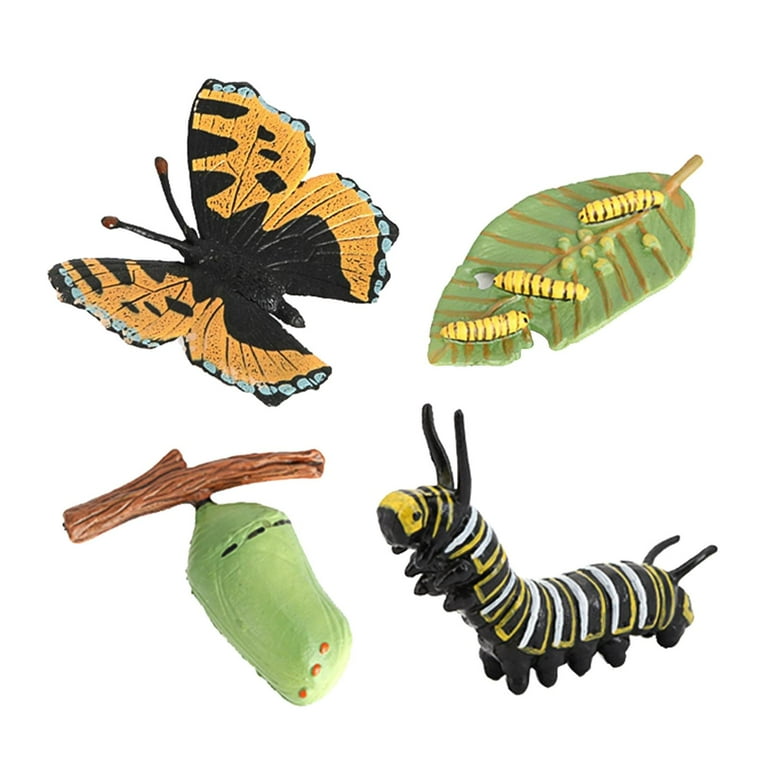This detailed image, set against a white background, showcases the fascinating metamorphic stages of a butterfly. In the upper left-hand corner, a striking yellow-orange butterfly with black central markings and intricate blue-ringed black edges on its wings is displayed with its wings spread wide. Centered on the right side is an illustration of a green and brown leaf, meticulously detailed with visible veins, supporting three small, worm-like yellow larvae. In the bottom left corner, a short branch extends with an oblong, green chrysalis, distinguished by three small cutouts at the top, hanging from it. To the right of this chrysalis is a vibrant caterpillar, predominantly black with yellow and white striations along its back and a vivid yellow face, poised with its head lifted. This composite image presents a comprehensive visual narrative of a butterfly's life cycle, from larvae and caterpillar stages, through the chrysalis phase, to its final stunning emergence as a butterfly.